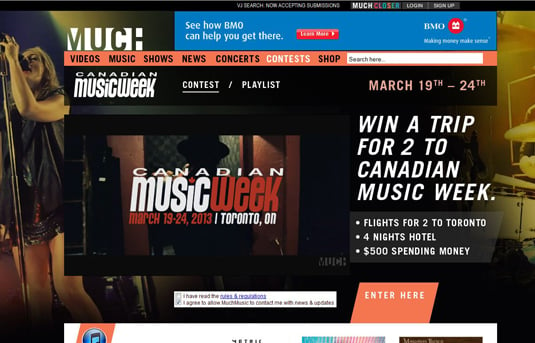The image features a dynamic scene with multiple elements. In the background, spanning both the left and right sides, is a blueish font that adds a sense of vibrancy. Dominating the foreground is a woman singing into a microphone, her passion evident as she performs. To her right, the faint outline of a drum set suggests she is part of a live performance.

At the top of the image, a black border with white text on the right side announces, "VJ Search Now Accepting Submissions." Below this, in a slightly darker white font, the word "Much" is displayed, followed by a multi-colored version of "Much" positioned closer to the viewer. Additionally, the options to "Login" and "Sign Up" are prominently available.

Midway down, the word "Much" appears outlined in white against an orangish-yellow background. Adjacent to this is an advertisement on a blue background. The ad, from a bank, features white text that reads, "See how BMO can help you get there," along with a red button and the BMO logo, which is a red circle with white detailing.

Beneath this, an orangish-colored section lists several categories— "Videos," "Music," "Shows," "News," "Concerts" (in white), "Contests," and "Shop"—in a mix of black and white text. 

Further down, a white search bar sits atop a black area filled with white text including "Canadian Music Week," "Contest," "Playlist." On the far right in gray text, dates "March 19th through the 24th" are displayed. A picture within this section highlights the main prize: a trip for two to Canadian Music Week, as detailed by big white text on the right.